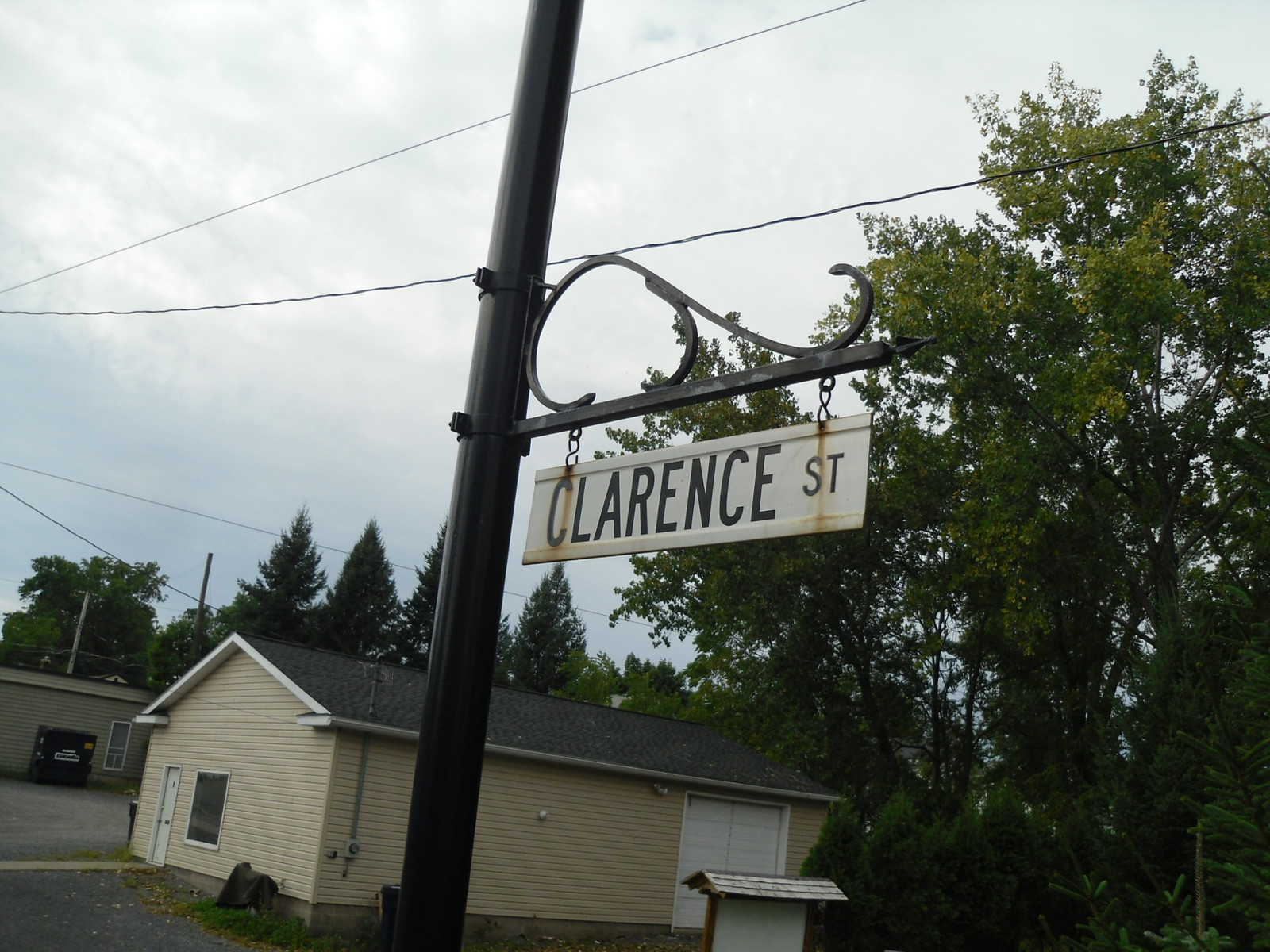This photograph captures a street sign for Clarence Street, mounted on a distinctive black pole featuring a wavy design element just above the sign. The street sign itself is rectangular with a white background and black font, suspended by short metal chains. Notably, there is some rust visible around the chains.

In the backdrop, a commercial-looking building made of light yellow material can be seen. This structure has a mix of features including a door, window, and a nearly solid wall with a vertical pipe running down it. Additionally, there are two large white doors to the right. Beyond this building, a similar type of structure and a dumpster are visible, indicating a possibly industrial or commercial area.

The scene is further enriched with natural elements; several trees are present, primarily to the right of the pole, along with more trees visible in the distant background. Power lines crisscross the sky, adding to the urban landscape feel of the photograph.